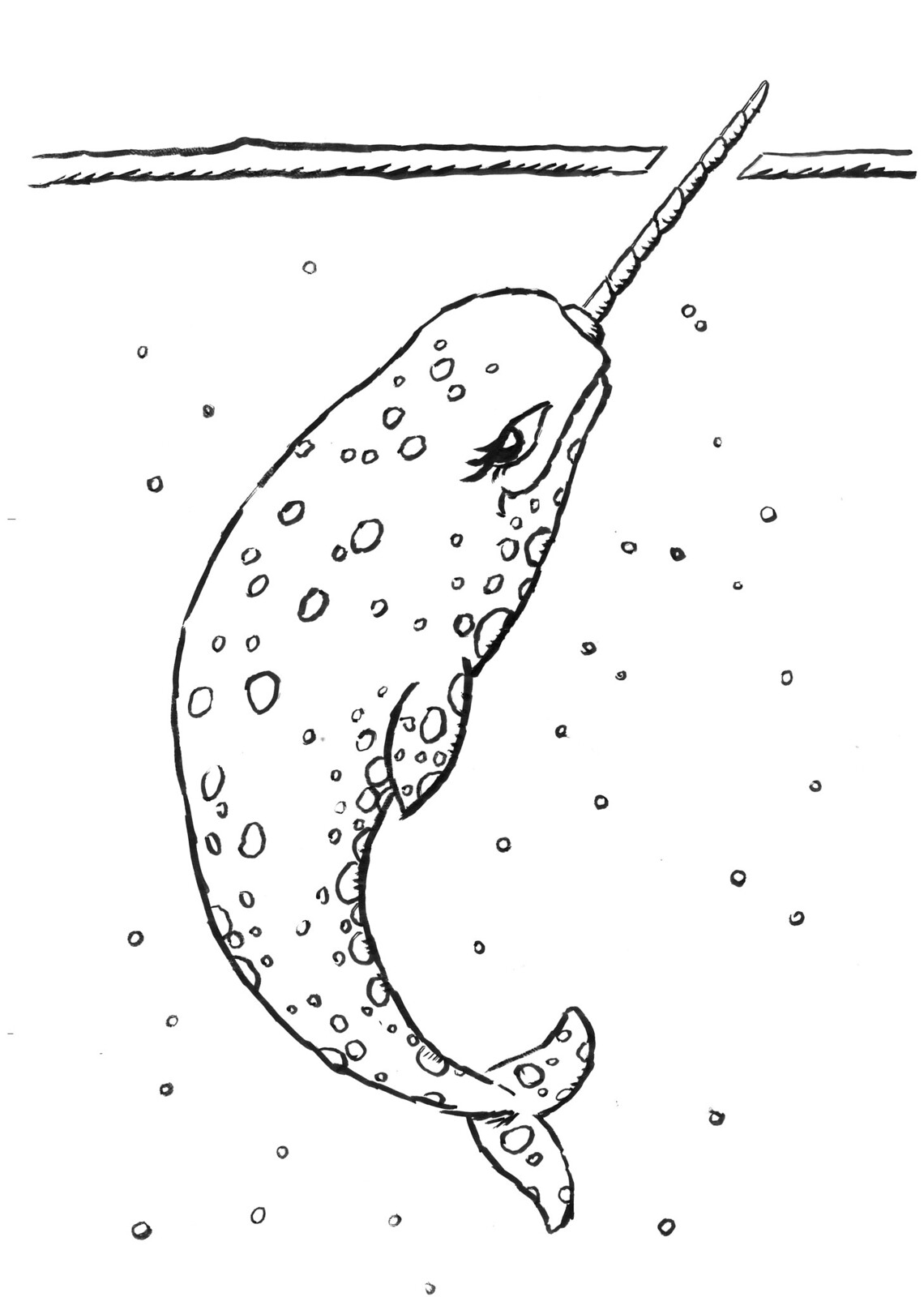The image is a detailed black-and-white drawing of a narwhal, shown from the right-side profile. The narwhal's body is adorned with numerous speckles or dots, and it features a small fin positioned in the middle of its body extending to the right. Its tail, located at the bottom right of the image, has two pointed fins that extend slightly up and down. A large, prominent eye is visible on the right side of the head, complete with eyelashes. 

A distinctive unicorn-like tusk or protrusion extends from the front of the narwhal's head, angling upwards and to the right. This tusk appears to puncture through a layer of ice at the top of the drawing, which is represented by two horizontal black lines with space between them, visually suggesting ice with water beneath. Bubbles are drawn around the narwhal, enhancing the underwater effect, while the entire scene is set against a plain white background. No additional coloring or shading is present, emphasizing the clean outline style of the drawing.